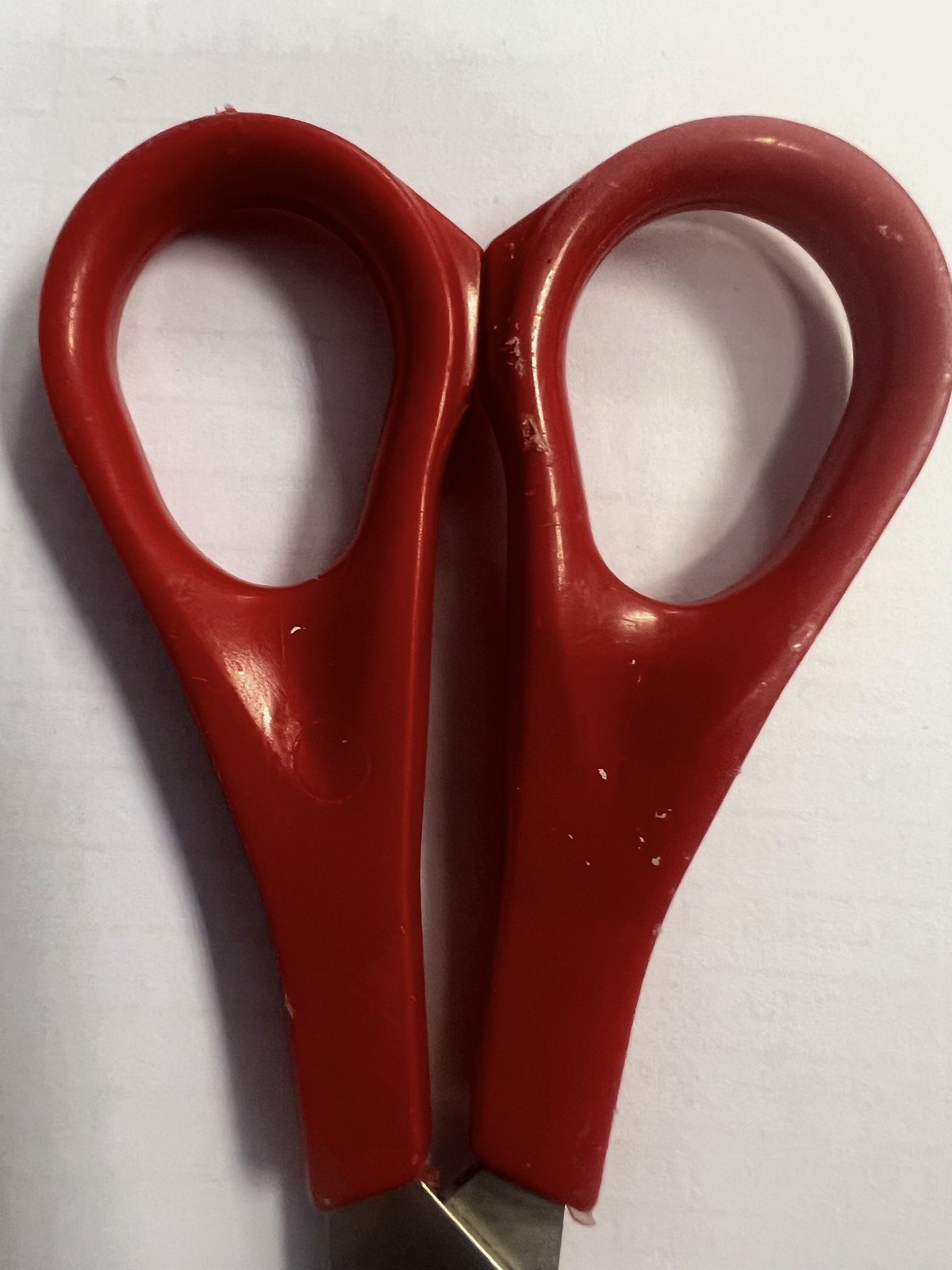This close-up photograph captures the handles of a well-used pair of scissors positioned vertically against a white background. The scissors feature plastic handles in a dark maroon or rusty red color, exhibiting clear signs of wear and tear, including dents, chips, and possible teeth marks. The background, mistaken for white paper, is actually composed of vertically arranged, rectangular white bricks. The metal part of the scissors below the handles is partially visible, casting a faint shadow on the background. The round cutouts in the handles, intended for finger placement, hint at the scissors' functionality amid their weathered appearance.